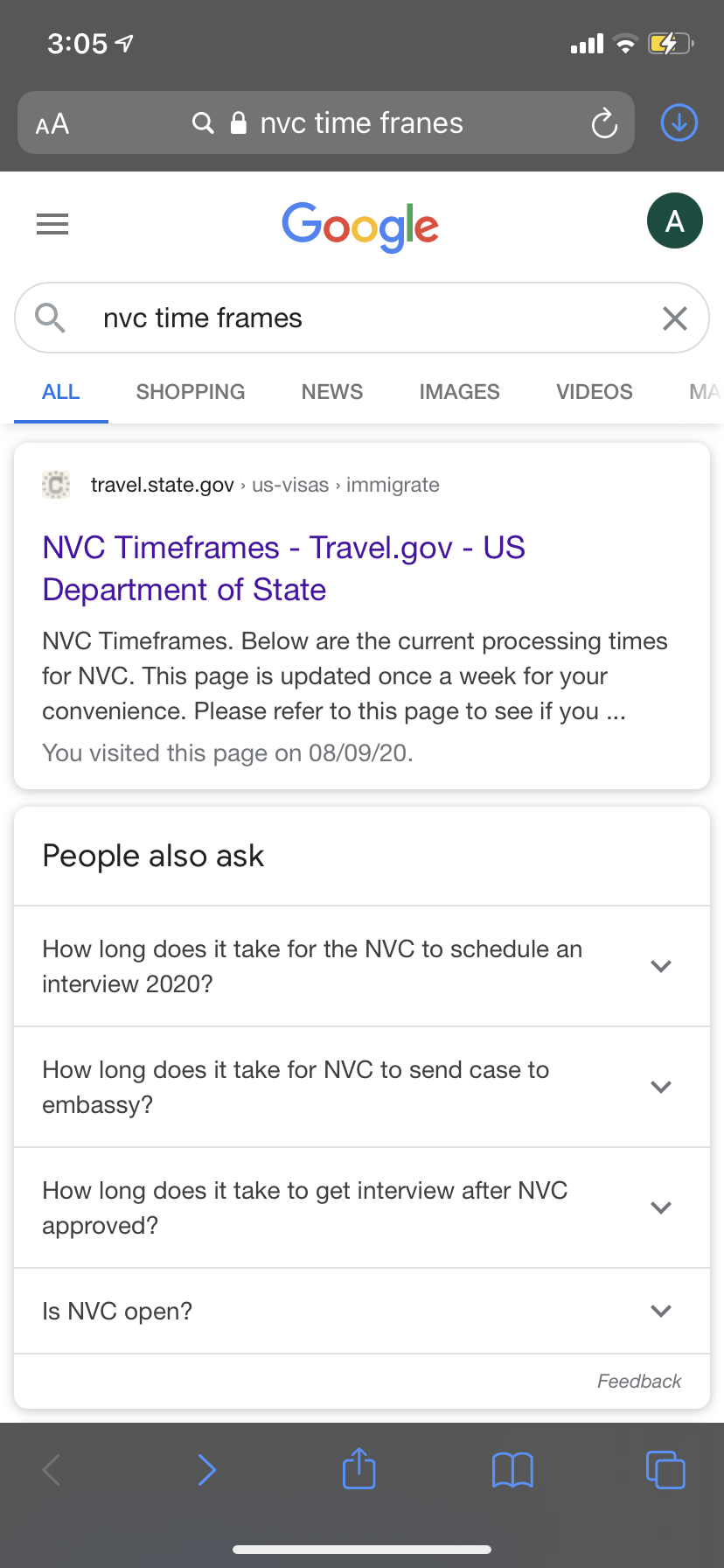The image is a screenshot of a Google search result, captured on a smartphone at 3:05 PM. The phone's status bar indicates a half-charged battery and a medium-strength service signal. 

At the top, the Google search query "NVC time frames" is prominently displayed, with the Google logo within the search bar. Below the search bar, the first result is from the travel.state.gov website, specifically from the US Department of State's Bureau of Consular Affairs. The site title, "NVC Time Frames," is followed by a brief description: "Below are the current processing times for NVC. This page is updated once a week for your convenience. Please refer to this page to see if you," with the text truncated at "travel...".

The screenshot also indicates that the page was visited on August 9, 2020. Further down, under the "People also ask" section, related questions are listed:
1. "How long does it take for the NVC to schedule an interview in 2020?"
2. "How long does it take for the NVC to send a case to embassy?"
3. "How long does it take to get an interview after NVC approved?"
4. "Is NVC open?"

At the bottom of the screen, options for sharing the search result or bookmarking the page are visible.